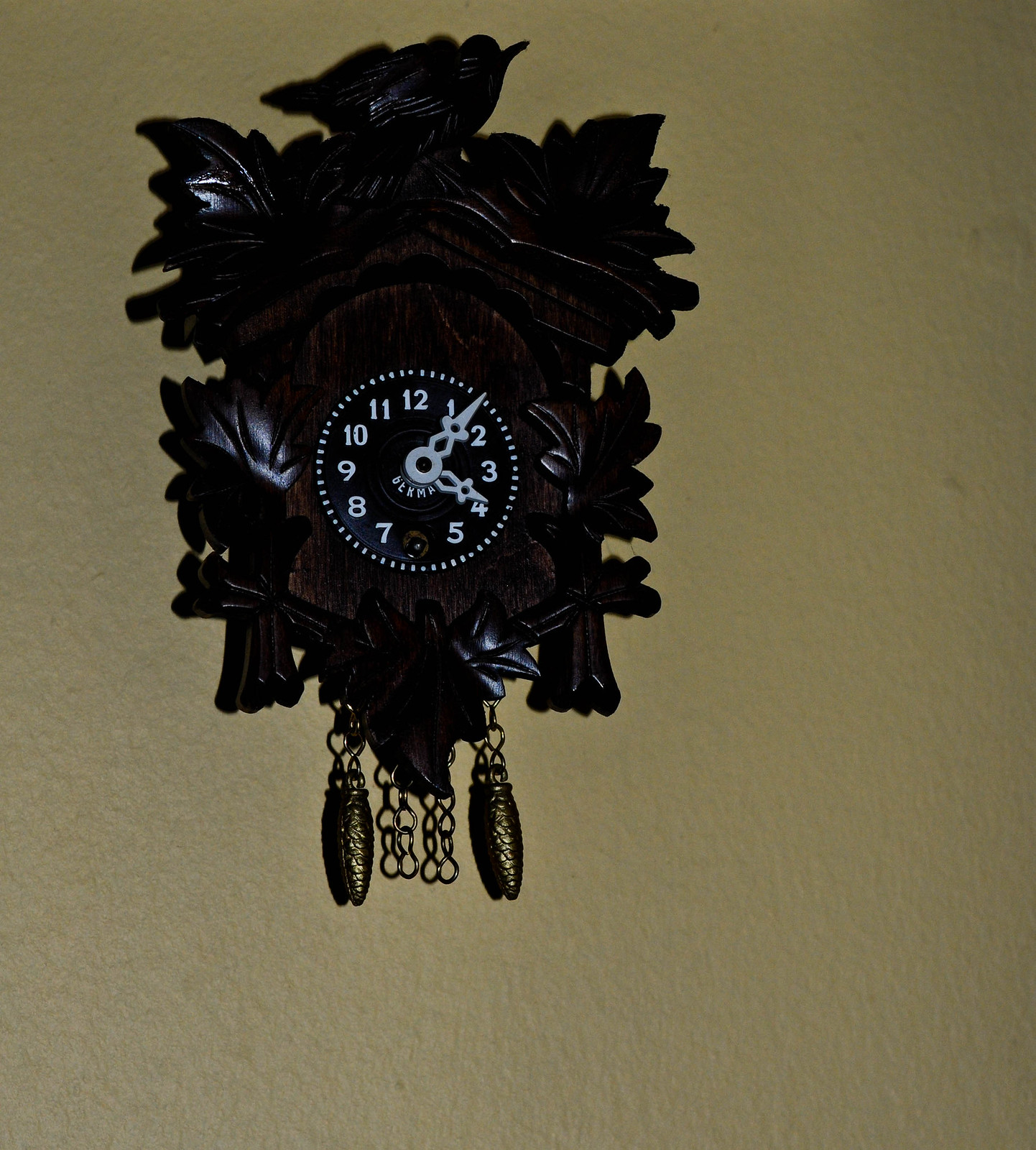This image features an intricately designed cuckoo clock, prominently displayed against a yellowish wall. The clock's circular dial, crafted from dark wood, showcases numbers from one to twelve, except for the number six, which is obscured by the winding mechanism. The clock's hands are a stark white, providing a striking contrast against the rich, dark background.

The entire structure is adorned with ornate carvings of leaves, illustrating an exceptional level of craftsmanship. At the very top of the clock sits a delicately carved bird, adding to the woodland theme. Suspended from the lower section are two metallic weights, likely serving as the pendulums essential for the clock's operation. Alongside these, a few chains are also visible, contributing to the clock's traditional aesthetic. This timeless piece brings a touch of rustic elegance to its surroundings.